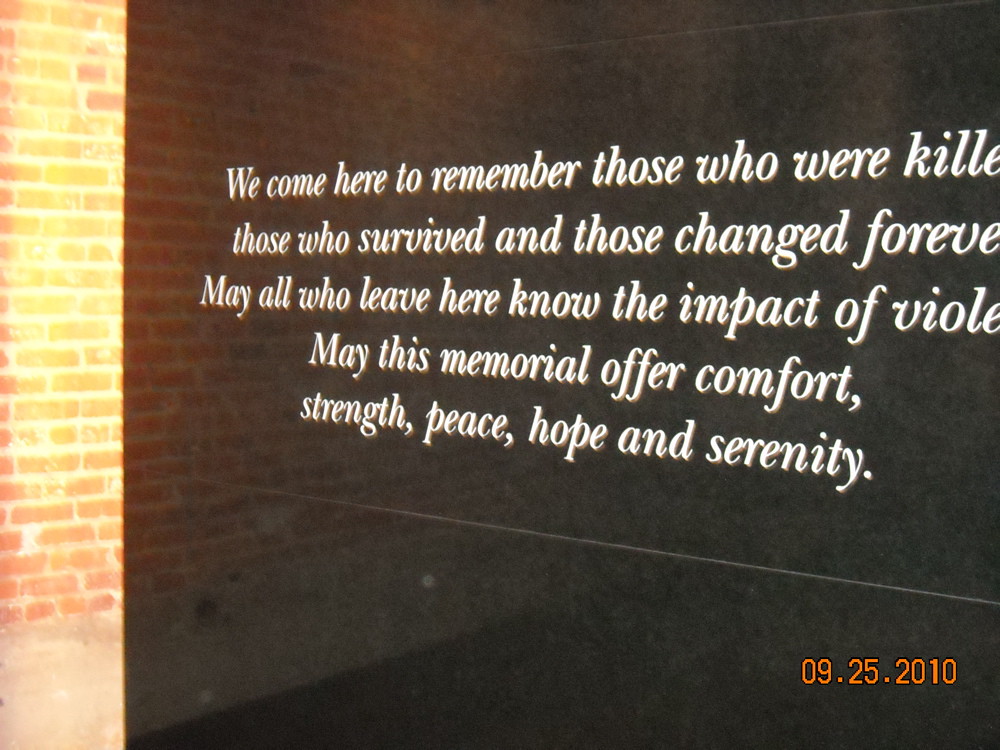This image is a photograph of a memorial plaque captured at an angle. The plaque is made of glossy black stone, featuring white text that reads, "We come here to remember those who were killed, those who survived, and those who were changed forever. May all who leave here know the impact of violence. May this memorial offer comfort, strength, peace, hope, and serenity." On the left side of the image, a red brick wall is illuminated by light, casting a reflection on the shiny black surface of the plaque. A small digital timestamp in red at the bottom right corner of the image reads, "09.25.2010."